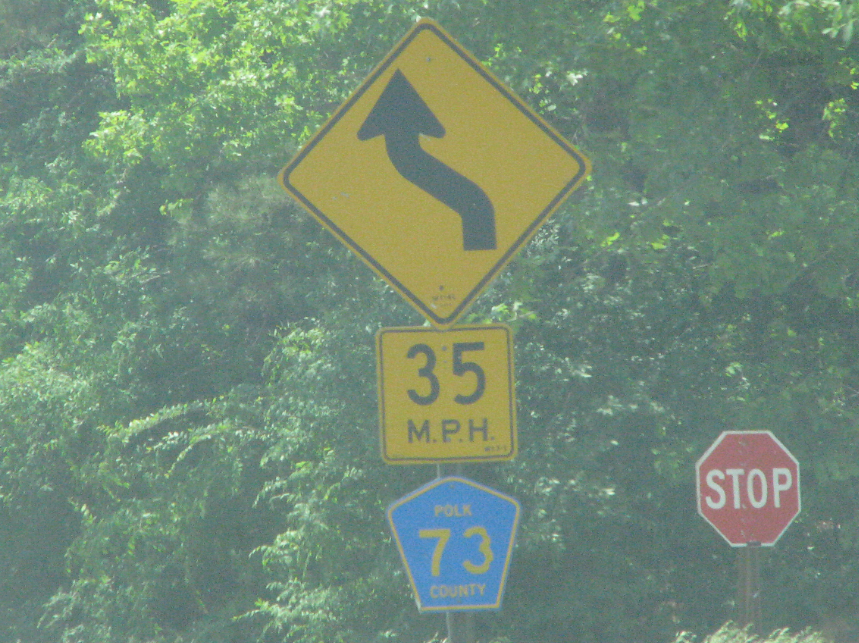This colour photograph, captured outdoors during the daytime, prominently features a series of road signs mounted on a single dark gray, circular pole positioned centrally in the image. The vibrant scene is set against a lush backdrop of dense green foliage, with sunlight streaming from the top left corner, contributing to a hazy glow across the scene. The pole displays three distinct signs from top to bottom. 

The top sign is a yellow diamond (oriented as a rotated square) with a black border, showcasing a black, double-curved arrow pointing upwards, indicating a winding road ahead. Below it, there is a smaller yellow square with rounded edges, bordered in black, bearing the number "35" followed by "M.P.H.," signifying a speed limit of 35 miles per hour. The third and lowest sign is pentagon-shaped with a blue background and a yellow border. It features the text "Polk" at the top, "73" in the middle, and "County" at the bottom, marking the boundary of Polk County.

To the right, slightly in the background, a traditional red stop sign with a white border on a rusty pole can be observed. The bottom of the image includes a hint of tall grass, completing the picturesque outdoor setting.